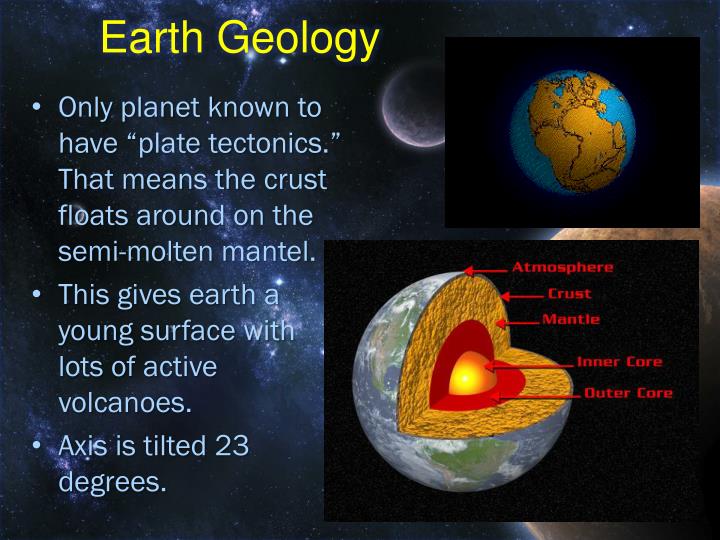The image, titled "Earth Geology" in prominent yellow letters against a dark gray, star-studded background, serves as an educational infographic about Earth's unique and dynamic geological features. On the left side, informative bullet points in white Times New Roman font detail the planet's distinctiveness: Earth is the only known planet with plate tectonics, meaning its crust floats on a semi-molten mantle, resulting in a youthful surface dotted with active volcanoes, and its axis is tilted at 23 degrees. 

The top right features a globe showcasing the Earth, displaying continents as if they were still part of a singular, ancient landmass. Below this, another graphic offers a cutaway view of the Earth's internal layers: a vibrant yellow inner core, a red outer core, a brownish mantle, gray crust, and a grayish-green-and-white atmosphere, all labeled with red text and arrows. This visually compelling poster encapsulates the dynamic and layered nature of Earth's geological structure.